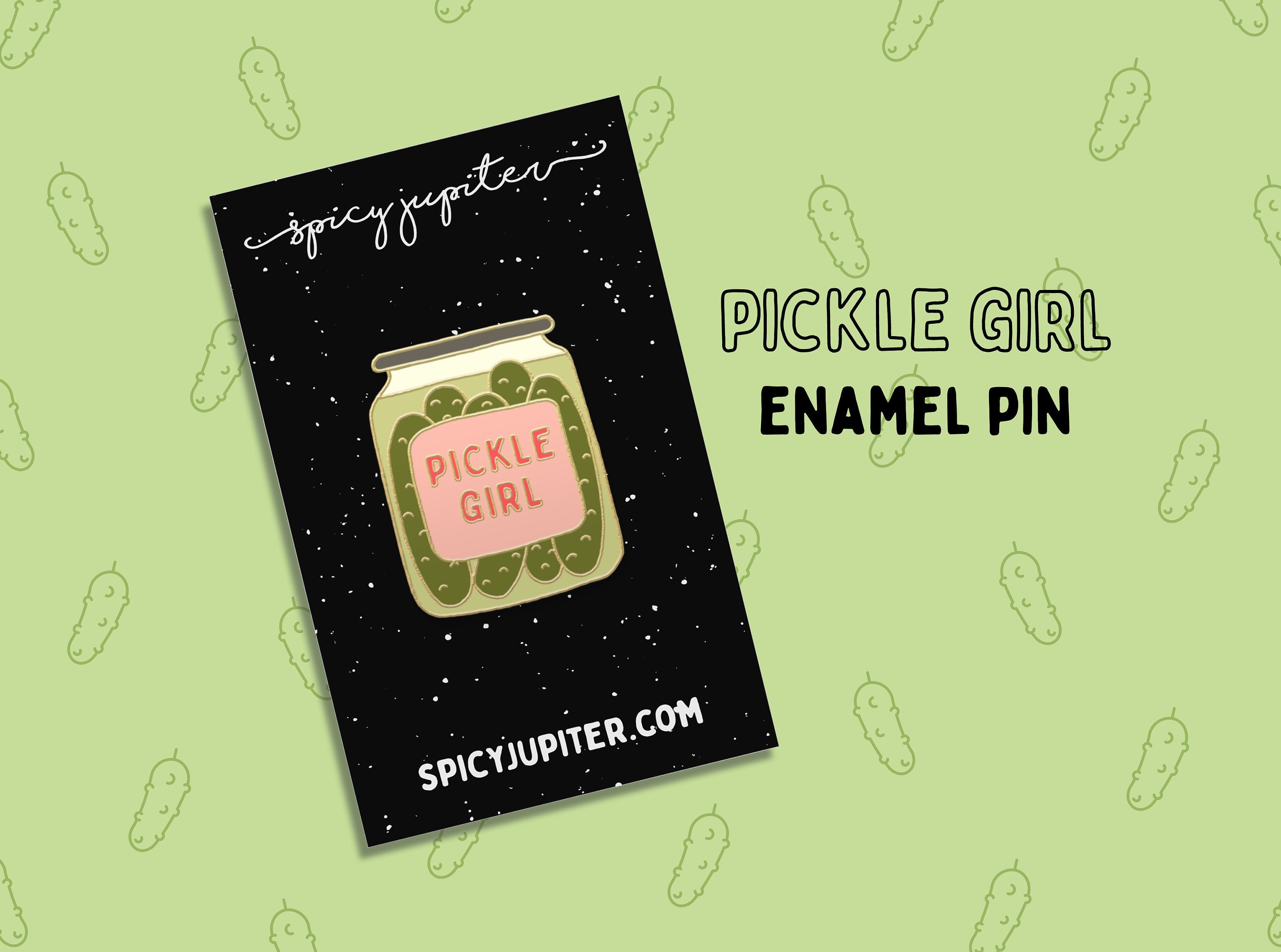This image features a vibrant advertisement set against a light green background adorned with scattered, darker green pickle illustrations, marked by crescent shapes to mimic pickle texture. Prominently, towards the left, is a black book cover speckled with tiny white stars. At the top of the cover, "Spicy Jupiter" is written in elegant cursive. Central to the cover is a drawing of a pickle jar labeled "Pickle Girl" on a pink label. Below this, the URL "spicyjupiter.com" is stated in bold, white capital letters. To the right of the jar, the text "Pickle Girl" appears in black bubble letters, with "enamel pin" in all caps below it, indicating the product being advertised.